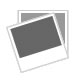The image depicts the back cover of a book, characterized by a predominantly brown background. On the left-hand side, there is a detailed illustration of a man and a woman, both dressed in 1950s-style attire. The man, facing the viewer, is dressed in a black and white pinstripe suit with a white tie and black shoes, topped with a gray fedora featuring a black ribbon. The woman, positioned to his left and facing him, wears a headband typical of the era, a mustard yellow shirt, a black skirt that falls above her knees, and black high heels. Her right hand reaches up towards the man’s chest.

At the top of the cover, a yellow text reads, "Roll right off the boardwalk through the peepholes and into the backroom bars." Below this, the author’s name, "Kuei Lin Lum," is displayed in orange text. A smaller text below introduces the book as a "paper doll passport through the constraints of prohibition," though the rest of the writing is difficult to decipher. The bottom right-hand corner features a couple of barcodes and a QR code for purchasing the book.